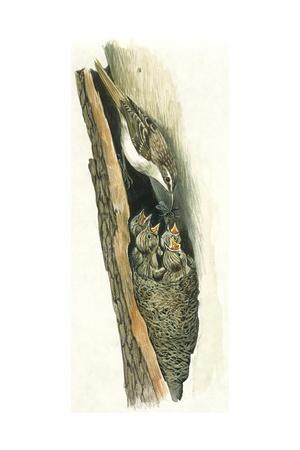This highly detailed, old-timey drawing illustrates a bird's nest ingeniously built inside a decayed hollow of a tree trunk. The background, a muted cream, highlights the tree with some of its bark stripped back, revealing a narrow entrance leading to a secluded tunnel, nestled safely between the bark and the tree. At the bottom of this tunnel lies the nest, meticulously woven from straw or moss, and shaped like a cone. Within this tightly packed nest, four baby birds eagerly await their meal, their beaks wide open and upstretched. Above them, the mother bird, with a tawny brown and tan plumage, and a characteristic white stripe above her eyes, leans into the hollow. She has a white underside and carries a small collection of worms in her beak, preparing to feed her anxious chicks. The image, devoid of any background distractions, focuses on this intimate and secluded moment, providing a close-up, almost x-ray-like view into the secret life within the tree trunk.